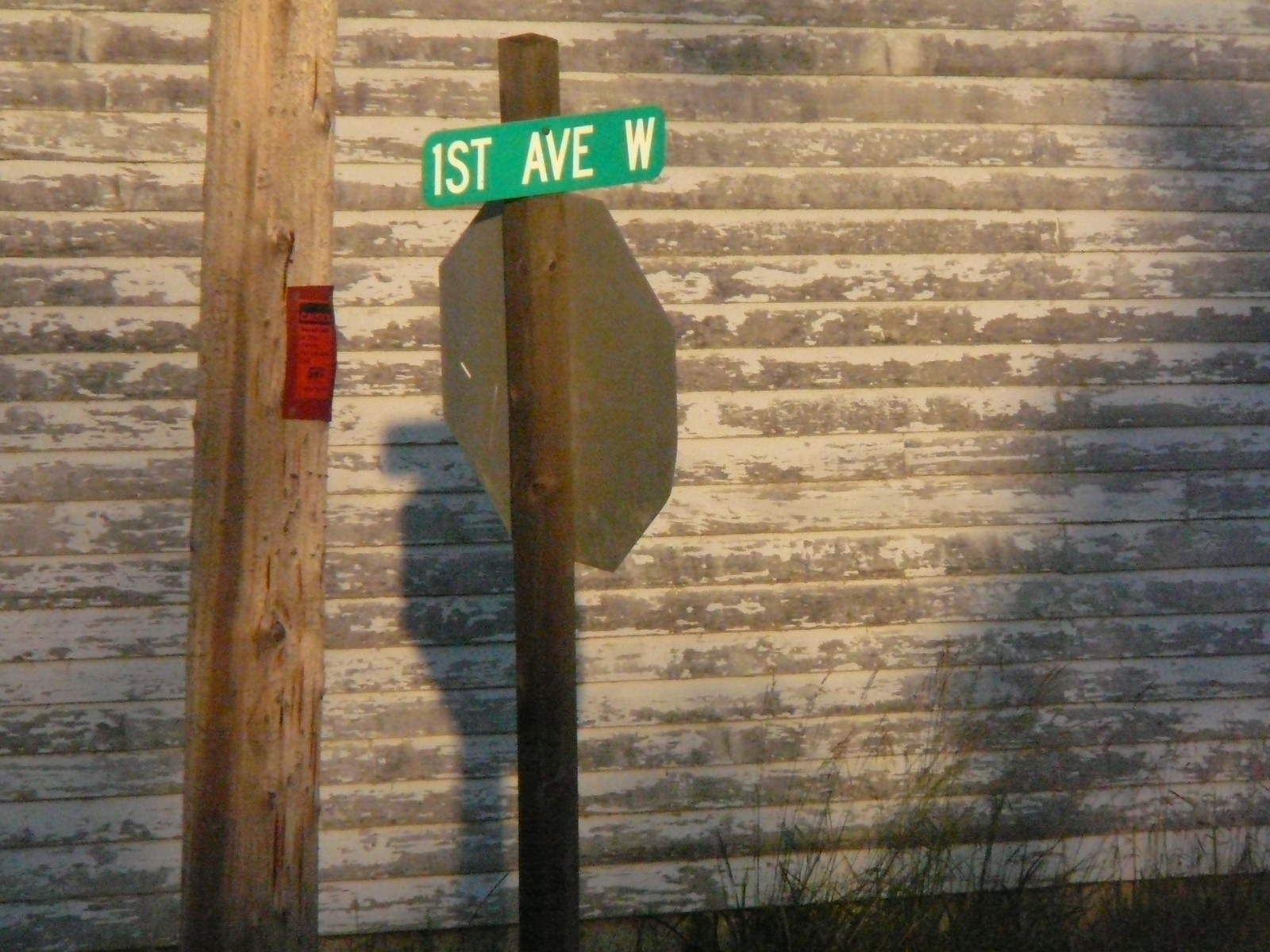This image shows a dilapidated side of a building with white siding, interspersed with areas of exposed gray where the siding has peeled off over time. On the left side of the photograph stands a tall, natural wood-colored telephone pole extending from the top to the bottom of the image. Near the center of this pole is a small, red rectangular sign, approximately an inch and a half tall, possibly stapled onto the wood. In the foreground, there's the back view of an octagonal stop sign, mounted on a long, dark brown pole. Attached near the top of the same pole is a green street sign with white capital letters reading "1st AVE W." The visible ground in the bottom right corner shows some scraggly grass growing adjacent to the building, lending an overall sense of age and disrepair to the scene.